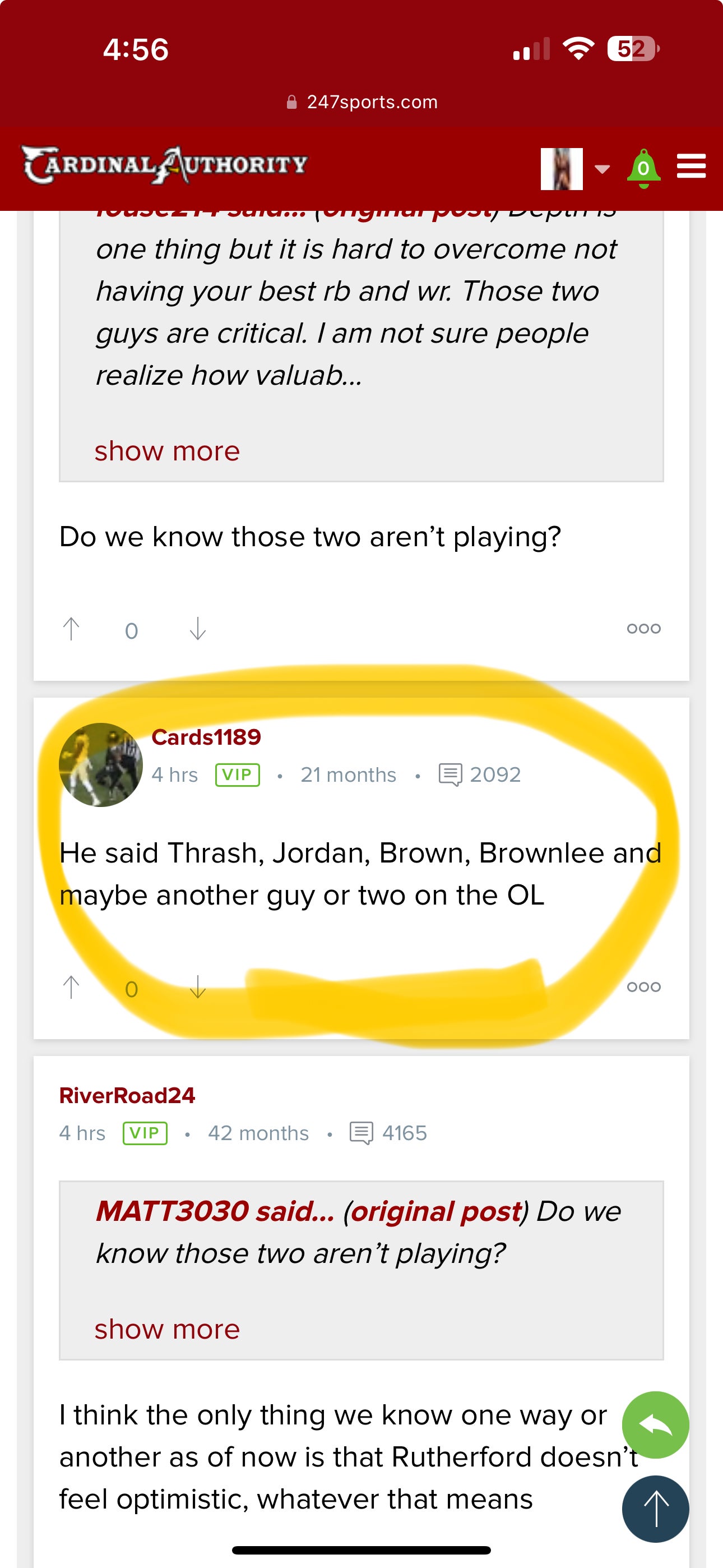This is a screenshot of a mobile phone interface displaying a webpage from 247sports.com. At the very top, the status bar has a red background, showing the time "4:56" on the top left. On the top right, indicators display a cell phone signal with two bars, a WiFi signal, and a battery icon at 52%, which is half full.

Below the status bar, the webpage details start with the website's name "247sports.com" accompanied by a lock icon, indicating a secure connection. The header of the website, titled "Cardinal Authority," is prominently displayed in red text.

To the right of the header, there is a white box containing an image, a green notification bell icon, and a hamburger menu button for additional options. Below the header, the webpage appears to be a social media feed. It includes several content boxes, each with profile information, text, and interaction icons.

One of the content boxes is highlighted with a yellow circle. Inside this white box, it shows a profile picture placeholder labeled "Cards 189," with details such as "4 hours" and "VIP" in a green box. It also mentions "21 months," adjacent to a chat bubble icon displaying "2092" comments. The post text below reads: "He said Thresh, Jordan, Brown, Brownlee and maybe another guy or two on the O line."

Another similar white content box is present below it, featuring additional user names and content. At the bottom right of the screen, there is a green circle with a left-pointing arrow, and beneath it, a blue circle with an upward-pointing arrow, likely for navigation purposes.